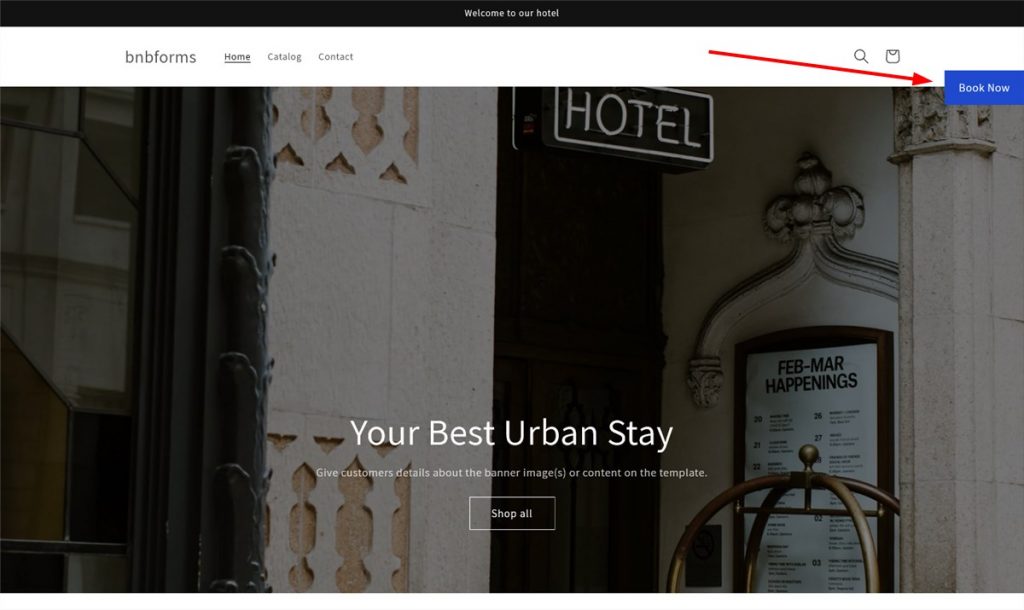This detailed caption provides a clear description of the screenshot for a company's urban stay website:

---

The screenshot displays the homepage of a website for a company specializing in urban stays. At the very top, a narrow black bar stretches across the screen with a welcoming message in small white letters: "Welcome to Our Hotel." Directly below this, a wider white bar contains the navigation menu, which includes links labeled "B&B Forms," "Home," "Catalog," and "Contact." The "Home" link is underlined, indicating the current page. To the right of these links, a search bar and a message icon are placed next to a blue rectangle button labeled "Book Now," highlighted by a red arrow.

The main portion of the screenshot showcases an image of the front facade of the hotel. The hotel's exterior is adorned with an old-fashioned sign that appears designed to light up, although it is unlit in this image. To the right of the entrance, an event sign is mounted, titled "February to March Happenings," listing several dates: 20, 21, 22, 26, 27, 28, and finally 02 and 03 at the bottom, though the specific events for each date are not readable. Various walls and pillars add architectural interest to the scene.

Overlaying the image in bold text is the slogan, "Your Best Urban Stay," suggesting an exceptional lodging experience. The banner encourages visitors to explore the website further, advising them to "Give customers details about the banner, images, or content on the template," and offering an invitation to "Shop All."

---
This caption provides a thorough and visually descriptive overview of the screenshot, allowing readers to easily visualize and understand the website's layout and content.